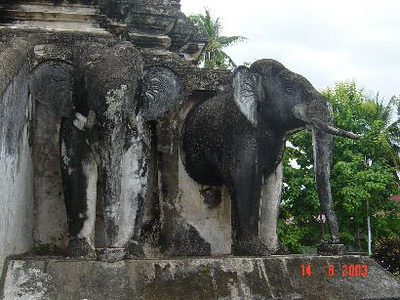This photograph, taken on August 14, 2003, captures a detailed stone sculpture of two elephants emerging from a wall. The statue, prominently featured in the center of the image, occupies about three-quarters of the frame. The elephants, one facing the camera head-on and the other in profile, are carved out of a weathered stone that displays various shades of gray and white due to aging and erosion. They appear to be coming out of a square enclosure, with their front halves extending outward.

The pedestal supporting the statue is constructed from the same stone and features stacked limestone, giving the impression of a substantial height, possibly around five feet. The sculpture exhibits a mixture of horizontal and vertical lines near its top left portion, suggestive of a pillar or some structural element.

In the background, leafy green trees and a patch of open sky provide a natural setting, with the tree predominantly occupying the right quarter of the image. The date "14-8-2003" is visibly printed in red text in the bottom right corner.